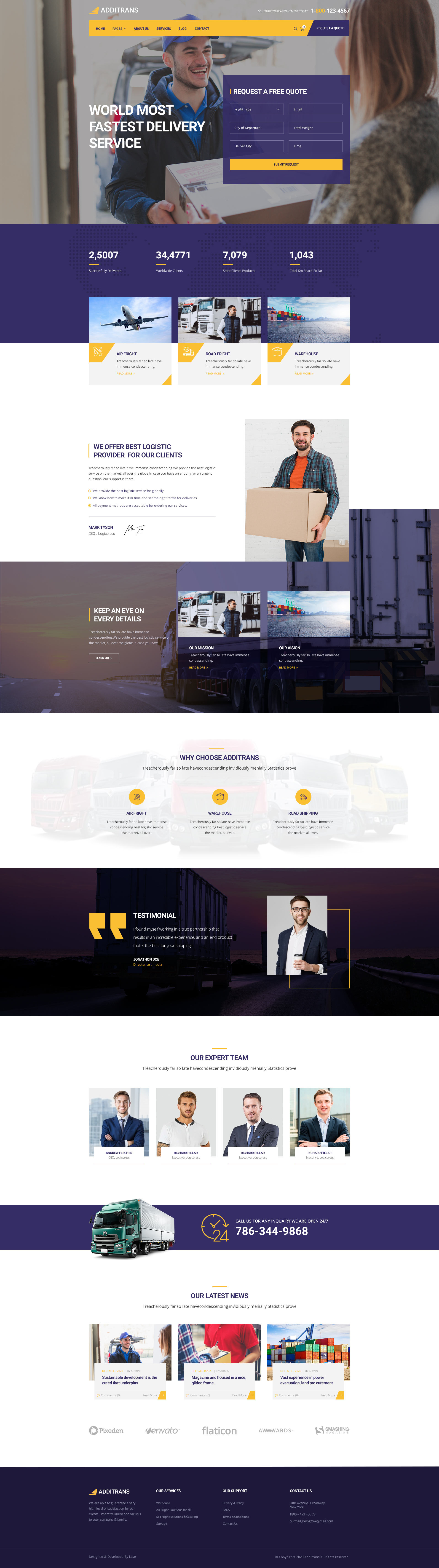Screenshot of Addytrans Website - Freight Delivery Service:

The screenshot displays the webpage of Addytrans, an online platform specializing in freight delivery services. The header section at the top of the page features a striking orange background with a comprehensive menu bar that includes options for Home, Pages, About Us, Services, Blog, and Contact. On the right side of this menu bar, there is a shopping cart icon and a Request a Quote button, which stands out with its purple background. Above this button, the contact number 1-800-123-4567 is prominently displayed.

Below the header, a functional purple box is situated, which facilitates users in requesting a freight quote. This box includes text fields for Freight Type, City of Departure, Delivery City, Time, Total Weight, and Email. At the bottom, an orange Submit Request button completes the form.

Adjacent to the purple box on the left, a bold white uppercase text asserts, "WORLD'S MOST FASTEST DELIVERY SERVICE." This section features a background image of a delivery person handing a parcel to a customer, enhancing the theme of prompt and reliable service.

Further down, a series of images depict the various services offered by the company, such as air freight, road freight, and warehousing. A testimonial from one of the directors is also included to provide potential clients with insights into the company's values and customer satisfaction measures.

At the bottom of the page, there is a group photograph of the company's executives, starting with Andrew Fletcher on the left and followed by others including Richard Pillar. Adjacent to this section, a purple banner featuring a telephone number (786-344-9868) and an image of a freight truck is prominently displayed.

The footer of the webpage includes a Latest News section showcasing three articles with accompanying images. The first article is titled, "Sustainable Development is the Creed that Underpins," the second reads, "Merit Magazine and House in a Nice Gilded Frame," and the third article states, "Fast Experience in Power Evacuation Land Procurement."

The very bottom of the footer provides essential information about Addytrans, covering sections such as Our Services, Our Support, and Contact Us, helping users navigate through various aspects of the company's offerings and assistance.

This detailed screenshot captures the comprehensive and user-friendly interface of Addytrans, emphasizing its commitment to fast, efficient, and diverse freight delivery solutions.